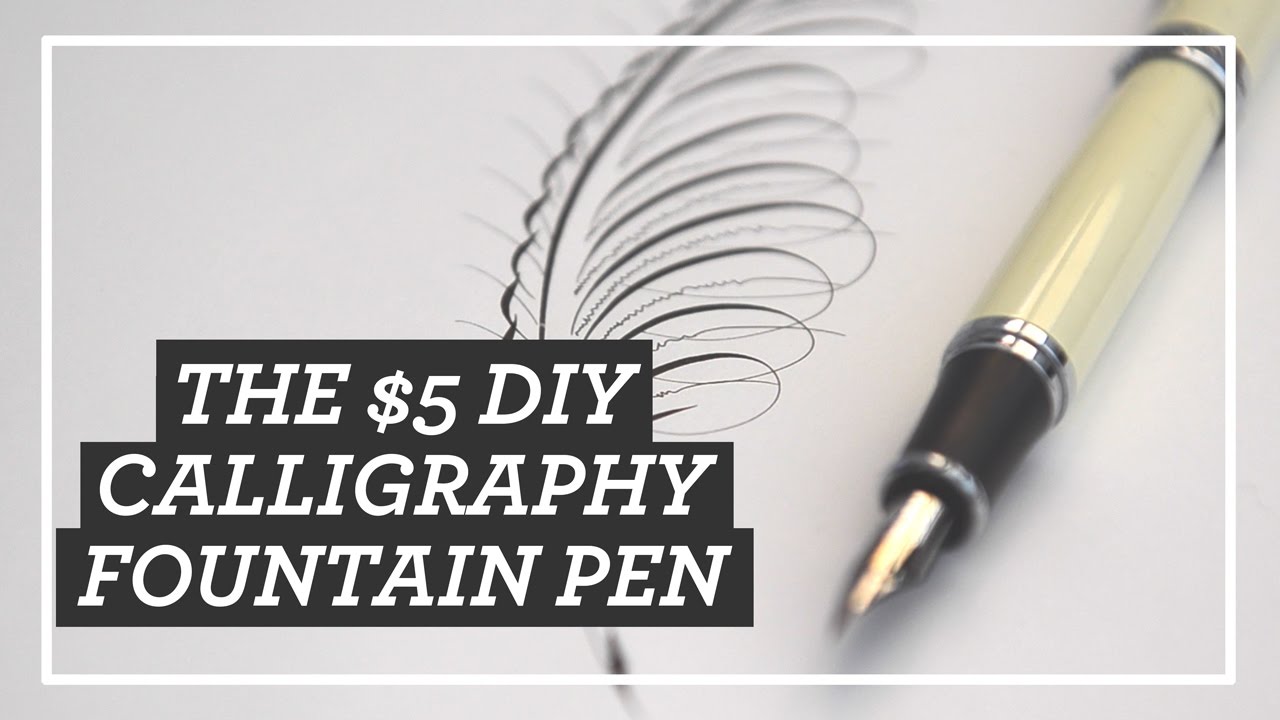The advertisement features a striking vertical photo with a grayish-white background that resembles a piece of paper. Central to the image is an elaborate black sketch of a feather, likely created with the advertised pen. Surrounding the photo is a white border that leaves a small margin where the background is visible, creating a framed effect. In bold white letters on a black rectangle overlay at the lower left, the text reads "The $5 DIY Calligraphy Fountain Pen," drawing attention to the product. The pen itself is diagonally positioned on the right side of the image. It has a pale yellow body with a black section near the bottom where the fingers would grip it and a tip that is a gray fountain pen point, though it is slightly blurred around the edges due to the resolution. The focus of the photo is primarily on the lower portion of the pen, with both the tip and the end of the pen slightly out of focus, adding depth to the image. This visually appealing and detailed composition effectively highlights the elegance and functionality of the calligraphy pen being advertised.